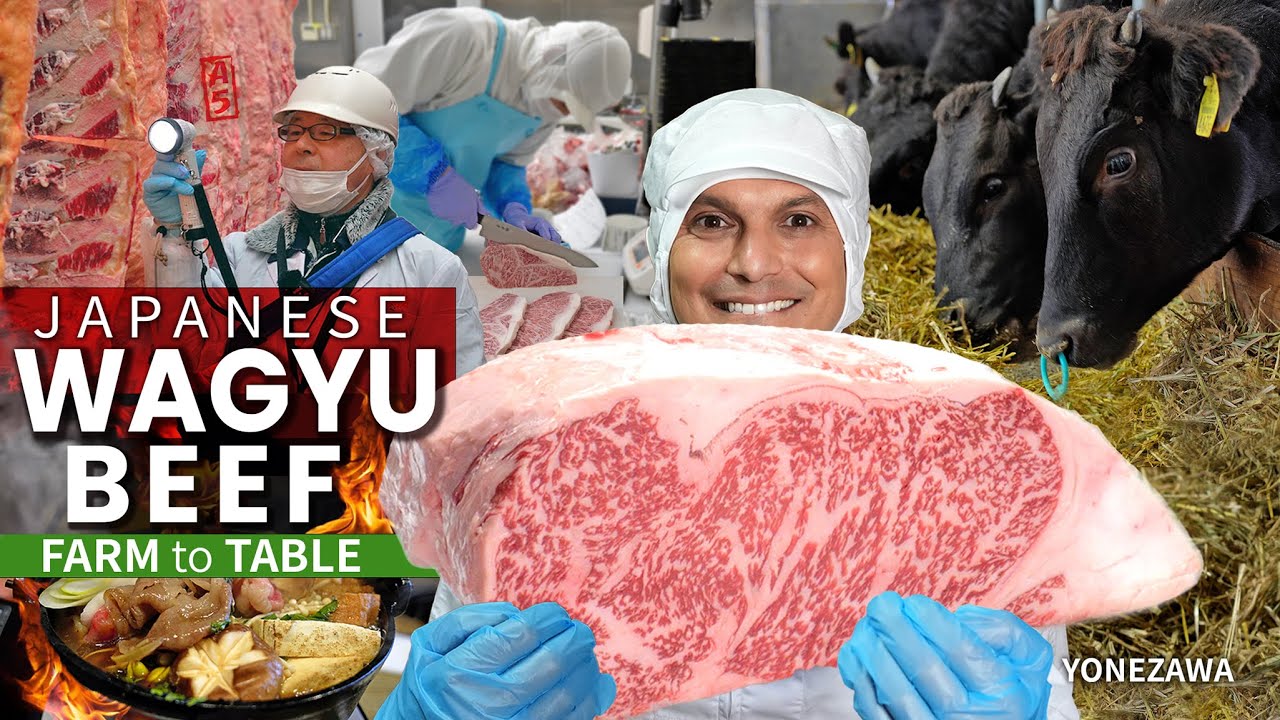The image titled "Japanese Wagyu Beef Farm-to-Table" showcases a complex scene at a meat processing facility. In the center, a smiling gentleman with an olive complexion is wearing a full white protective suit, including a head covering, and blue gloves. He proudly holds up an impressively large, marbled cut of Wagyu beef, characterized by its intricate patterns of red meat and white fat. In the background, to his right, a row of black cows is visible, some of which have nose rings and are feeding on hay. In the upper right corner, photographs of bulls or cows are displayed. To the left of the central figure, other workers, clad in similar white uniforms and blue aprons, are engaged in the butchering process, with one person using a flashlight. In the bottom left corner, a bowl of soup with various ingredients is presented, while on the bottom right, a watermark reads "Yonezawa." The top left corner of the image contains the text "Japanese Wagyu Beef: Farm-to-Table" next to a stylized depiction of food.